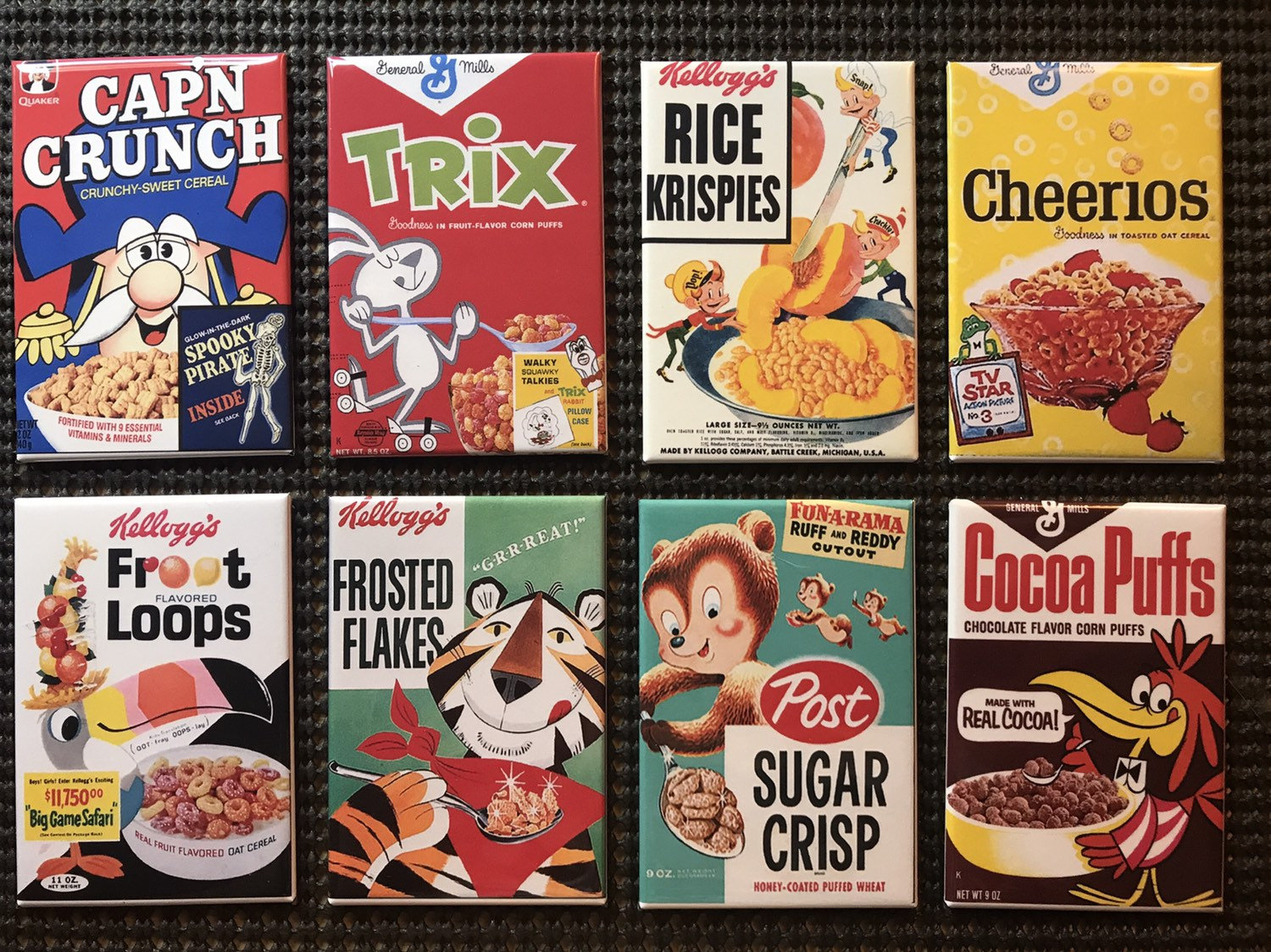This color photograph showcases a retro-themed collection of eight cereal box magnets from the 1960s or 1970s. Arranged in two rows of four against a dark brown, mesh-patterned surface, the magnets include detailed, three-dimensional artwork. The top row features Cap'n Crunch, Trix, Rice Krispies, and Cheerios, while the bottom row includes Froot Loops, Frosted Flakes, Sugar Crisp, and Cocoa Puffs. The vibrant colors—red, blue, yellow, green, pink, and brown—reflect the playful and nostalgic design of classic kid cereals. The magnets appear slightly curved along the edges, emphasizing their three-dimensional nature.